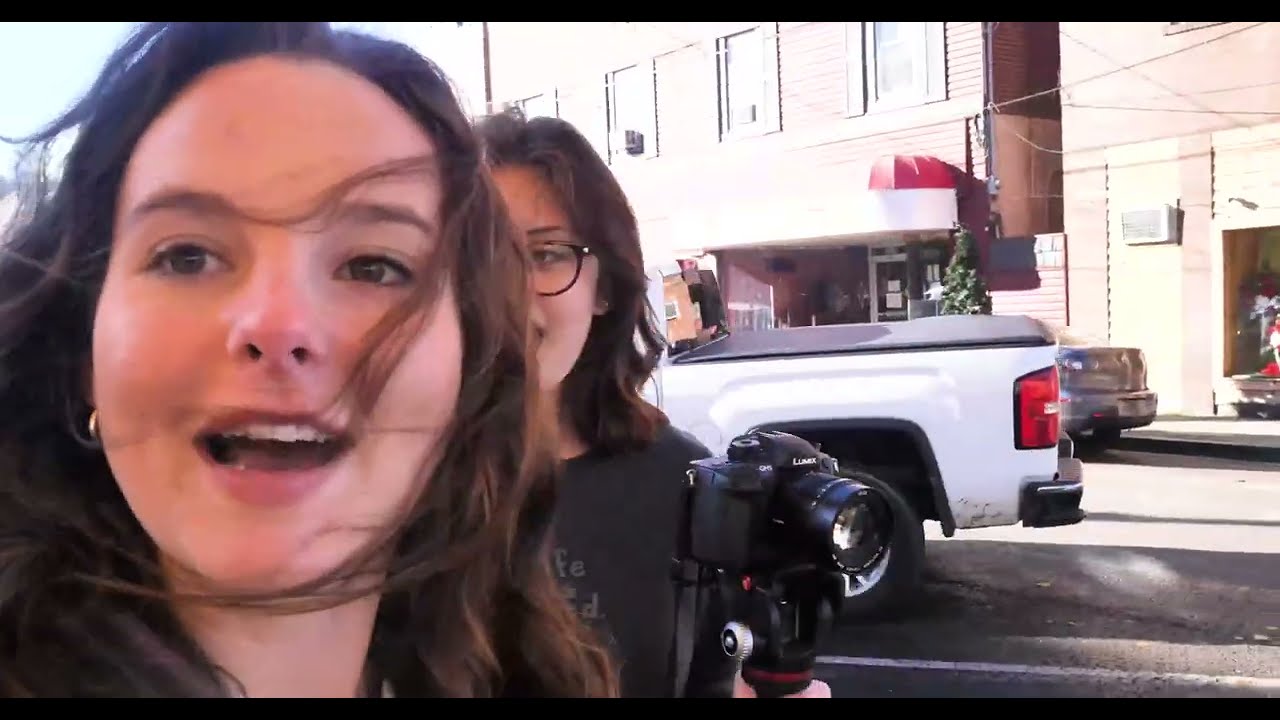The image captures a close-up, impromptu moment of two women with surprised expressions, seemingly taking a selfie or captured in a video frame. The woman in the foreground, with long, dark brown hair partially blown across her face by the wind, has brown eyes, is showing her top row of straight teeth as she talks animatedly, and wears small gold hoop earrings. The second woman, positioned slightly behind and to the right, has wavy dark brown hair with subtle gold highlights and is seen through large black-framed glasses. She holds a DSLR camera on a tripod, is wearing a black shirt with the partial text "Life is Good," and appears to be capturing the scene. The background reveals a sunny street scene with a glare from a bright light source. Parked on the street is a white truck with a covered bed and a silver car in front of a brick building with storefronts.